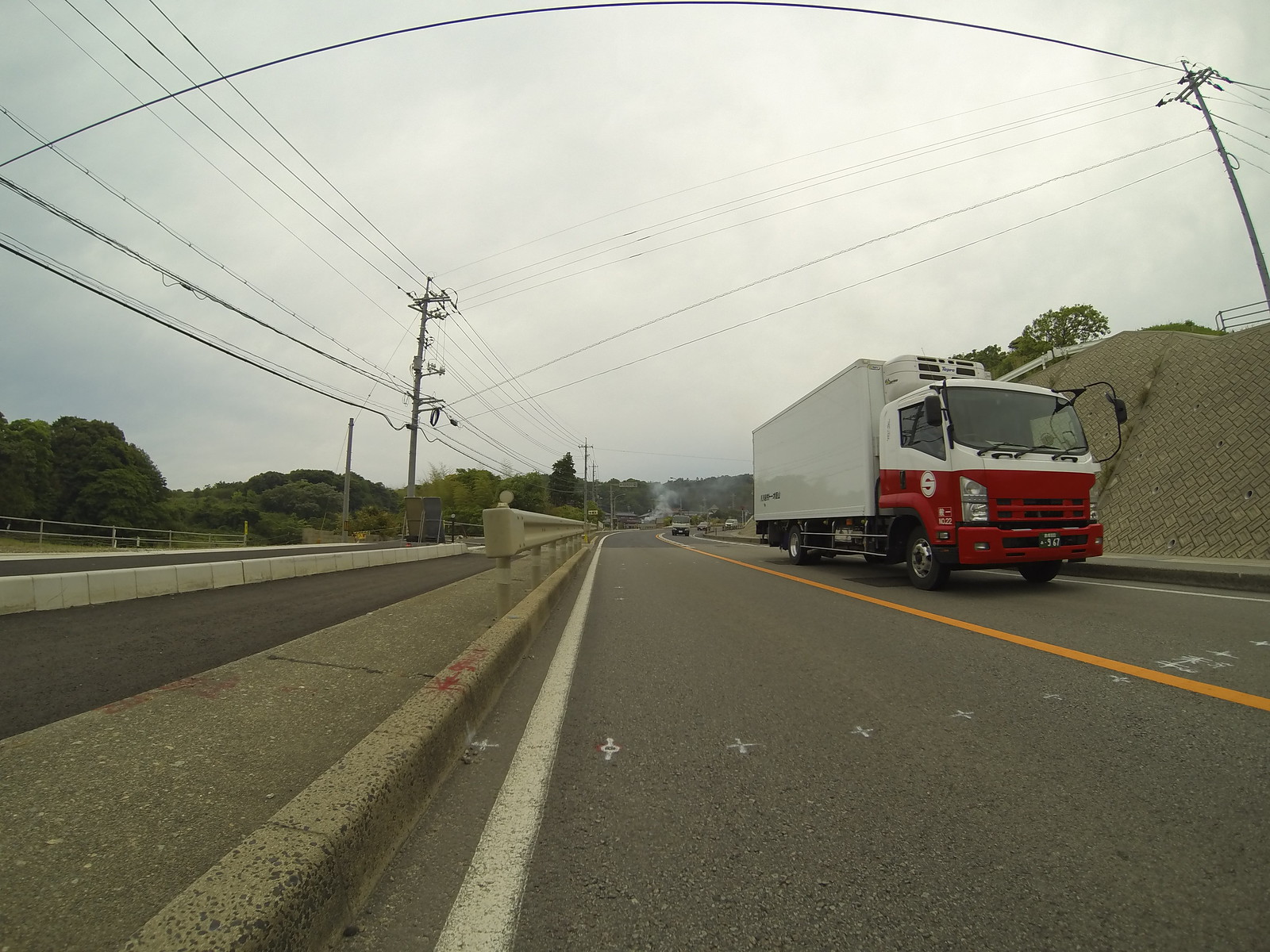A captivating real-life photograph captures a dynamic street view from an extremely low angle, creating the perspective that the camera is either sitting on the pavement or mounted on the back of a passing vehicle. Dominating the scene is a distinctive truck, its front half painted red on the lower section and white on the upper section, coupled with a white trailer. The image employs a fish-eye lens, introducing a notable curvature to the upper lines, where an electric pole and a web of electrical wires stretch across the frame.

To the right of the street, a brick wall topped with cement runs parallel to the roadway, adding texture and depth to the urban landscape. A solid yellow line bisects the asphalt, accompanied by various road markings. In the distance, a few cars are faintly visible, adding a sense of depth and continuity to the bustling street.

On the left side, a concrete divider separates the street from another road, while clusters of electric wires extend along the entire length of the scene. Behind them, the tops of numerous trees peek into the frame, their greenery contrasting with the urban setting. The sky above is overcast, lending a grayish hue to the daylight atmosphere, adding an element of dramatism to the photograph’s composition.